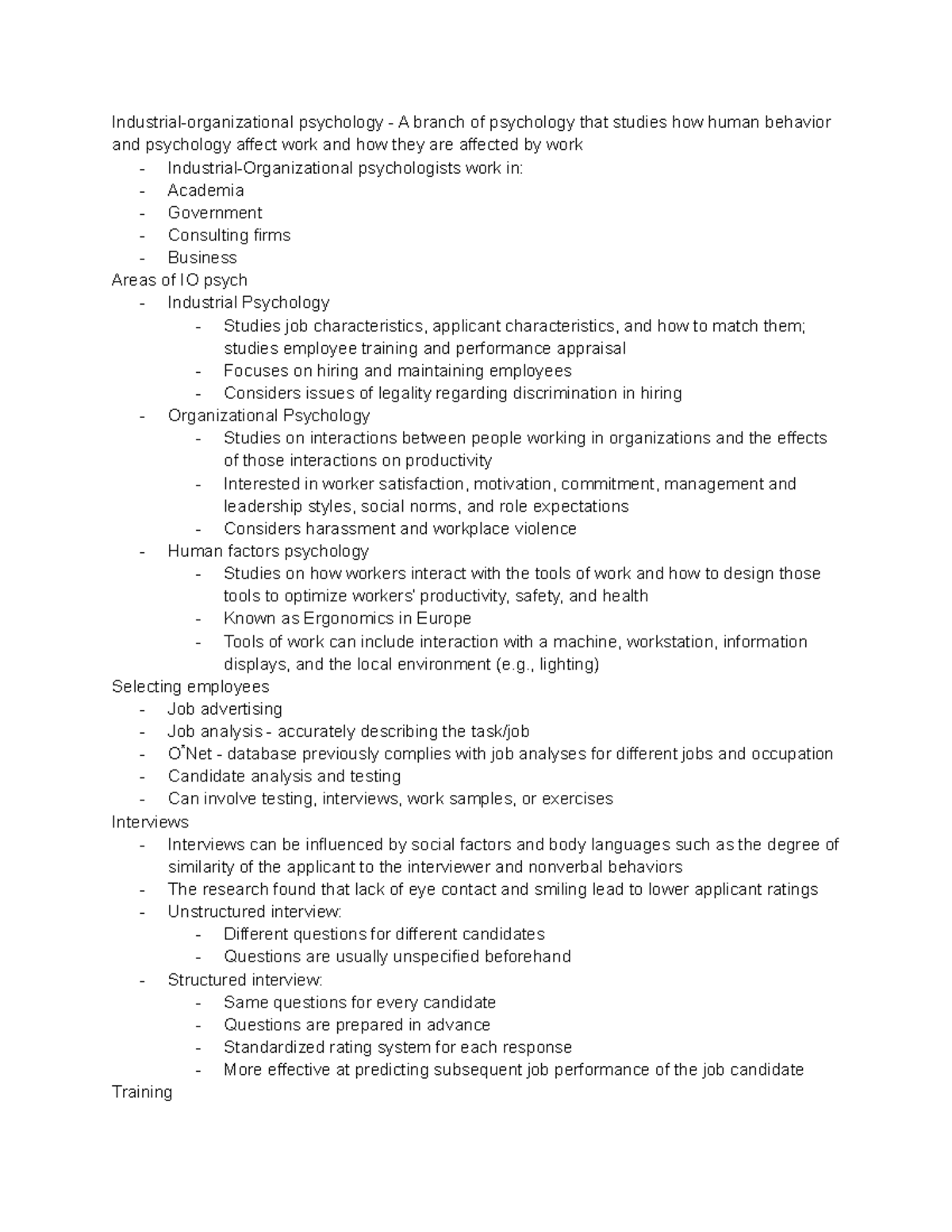This image features a document presented in portrait mode, with text in small, black font on a white background. The document contains eight paragraphs of text. 

At the top, there's a heading that reads: "Industrial-Organizational Psychology – a branch of psychology that studies how human behavior and psychology affect work and how they are affected by work."

Below the heading, a bulleted list explains where industrial-organizational psychologists often work:
- Academia
- Government
- Consulting firms
- Business

The next section starts without a space and is titled "Areas of I-O Psych:"
- Industrial psychology:
  - Studies job characteristics, applicant characteristics, and how to match them.
  - Studies employee training and performance appraisal.
  - Focuses on hiring and maintaining employees.
  - Considers issues of legality regarding discrimination in hiring.

The document continues with additional headings such as "Selecting Employees," "Interviews," and "Training" at the bottom.